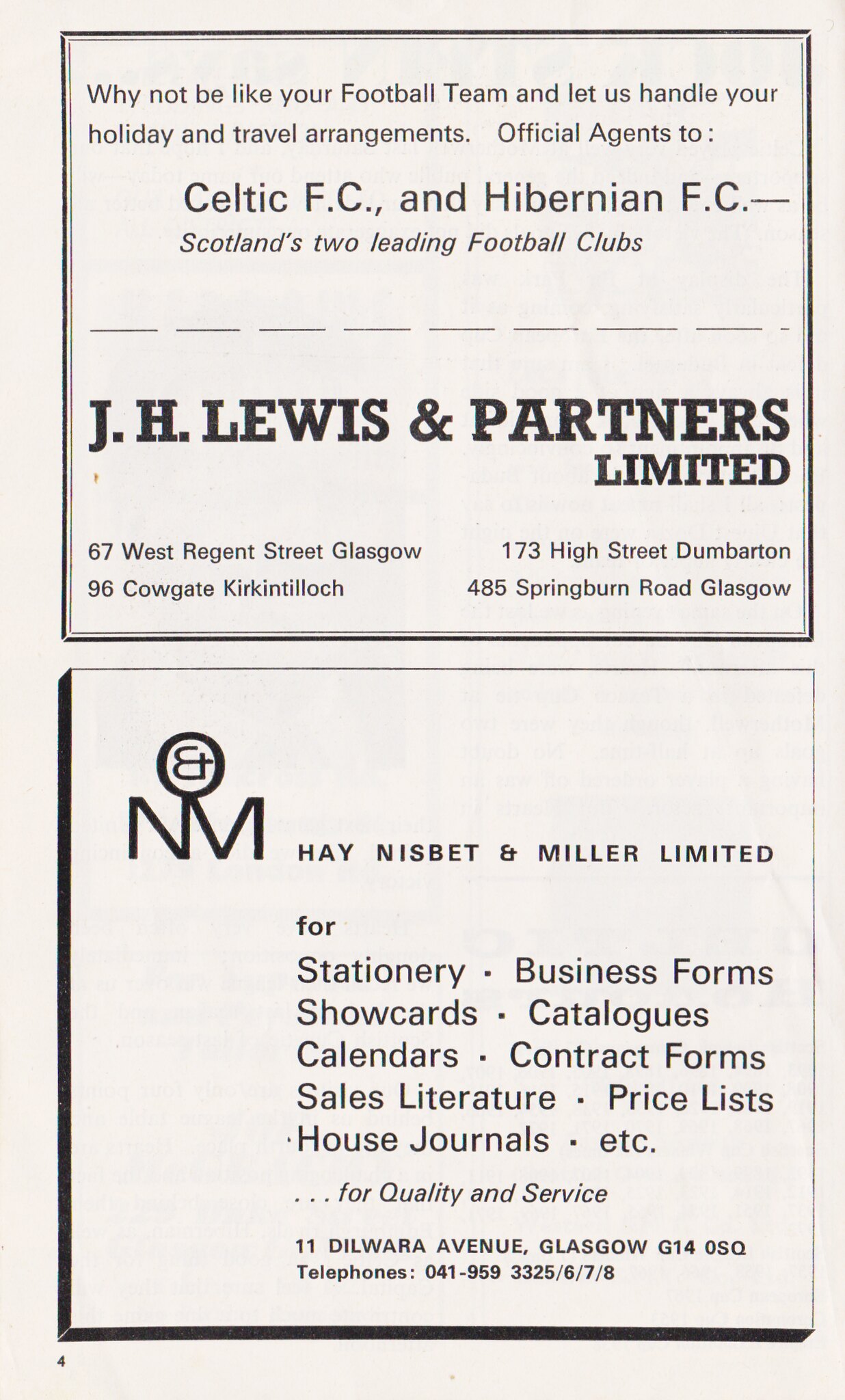The image is a page from a magazine, specifically page 4, as indicated by the number on the lower left corner. The page is divided into two black-bordered sections, each containing a distinct advertisement in black text. The top section promotes J.H. Lewis and Partners Ltd., highlighting their role as the official agents for Celtic FC and Hibernian FC, two leading football clubs in Scotland. Their services include handling holiday and travel arrangements, with offices located at 67 West Regent Street, Glasgow; 173 High Street, Dumbarton; 96 Cowgate, Kirkintilloch; and 485 Springburn Road, Glasgow. The bottom section features NM, Hay, Nisbet and Miller Ltd., emphasizing their wide range of products such as stationery, business forms, show cards, catalogs, calendars, contract forms, sales literature, price lists, and house journals. The advertisement guarantees quality service and provides their address at 11 Delaware Avenue, Glasgow G14 0SQ, along with contact telephone numbers 041 945 3325/6/7/8. A circular logo containing an ampersand (&) and the company's name accompanies this section.